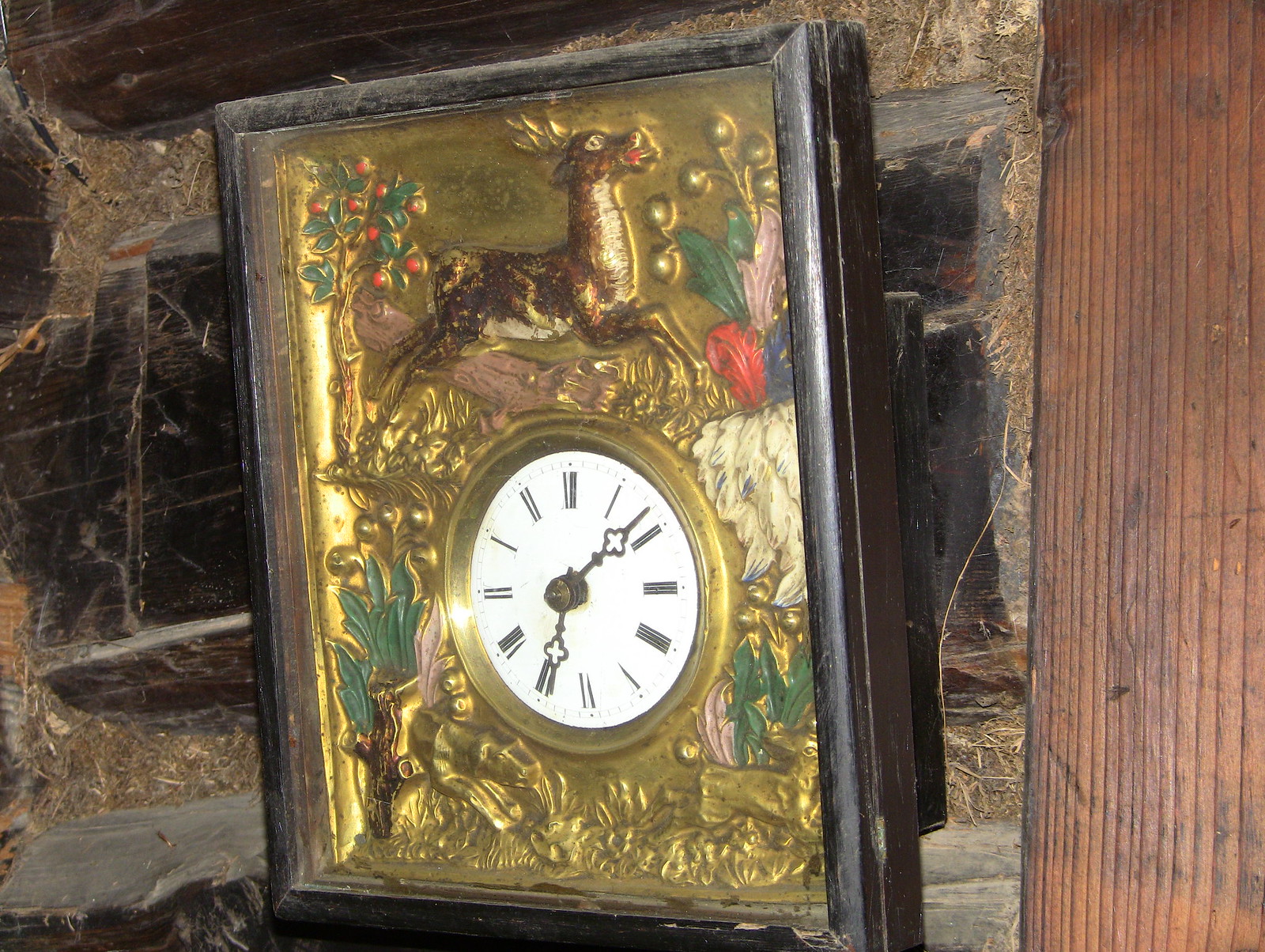A captivating photograph showcases a vintage framed clock resting against a rustic wooden wall. To the right, a wooden panel extends vertically, adorned with distinctive vertical indentation lines that add texture to the scene. The clock is set against an aged, possibly log wall, revealing the weathered allure of old wood. The clock itself is elegantly fashioned in gold, with its face featuring a serene depiction of a deer gracefully running through a field surrounded by trees bearing some kind of fruit. The clock's inlay is a pristine white, contrasting beautifully with its striking black hands. The time is marked by Roman numerals, and it appears to indicate 7:08.